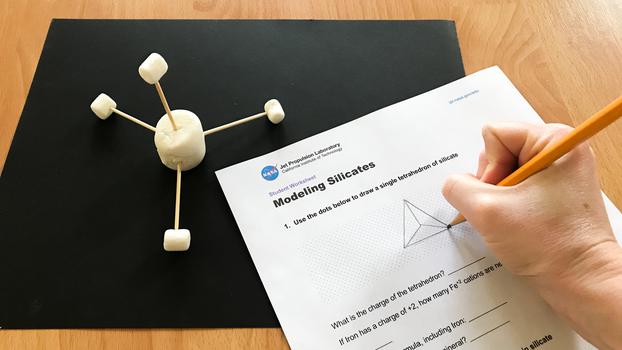The image depicts a light brown wooden desk or table, with a black rectangular sheet of paper on top. Centered on the black paper is a large chunky marshmallow with four toothpicks protruding from it, each tipped with a mini marshmallow. An individual holds an orange pencil and is drawing a triangle on a white sheet of paper. The paper is part of a student worksheet from NASA's Jet Propulsion Laboratory, titled "Modeling Silicates." The paper includes instructions to draw a single tetrahedron of silicate and contains further questions about the charge of the tetrahedron and iron cations. The text is in black against the white background, with an emblem and blue circle partially displayed at the top.